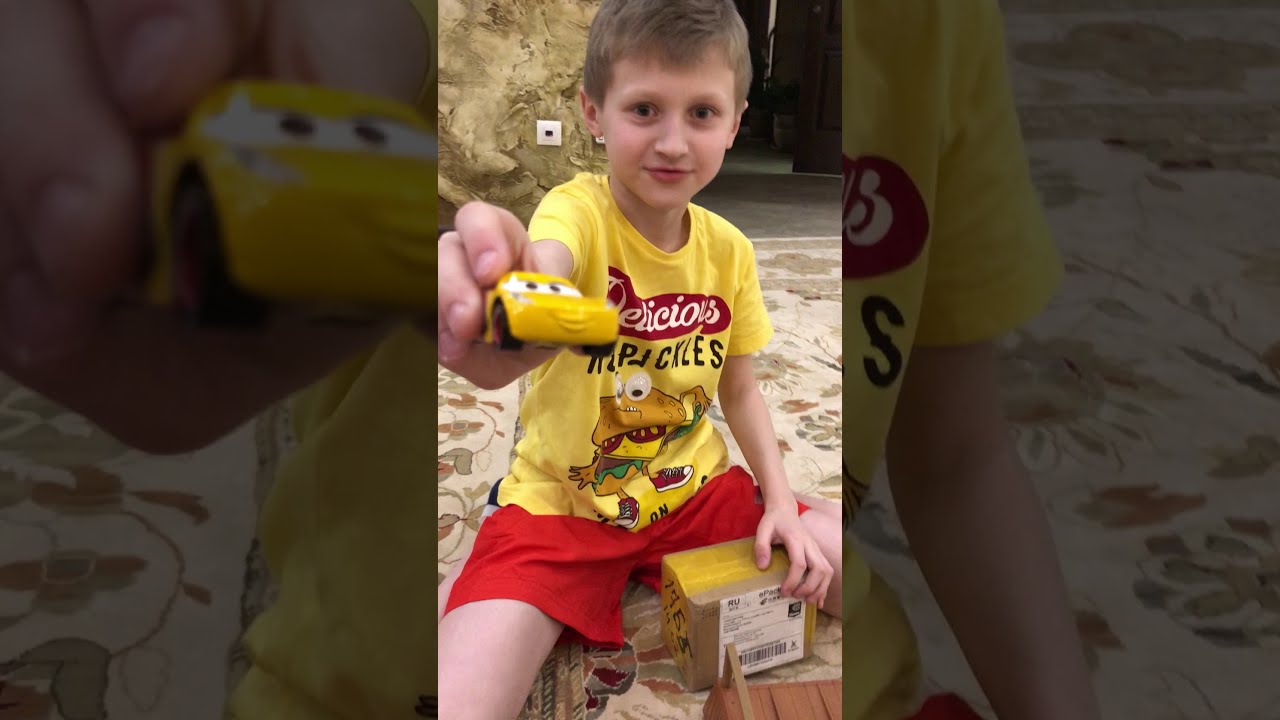The photograph, captured indoors in a living room, features a Caucasian boy of about five or six years old. The child, who has light brown hair and a subtle smile on his face, is dressed in a yellow t-shirt adorned with the animated figure of a sandwich wearing red sneakers and the words "Delicious Pickles." He also wears red shorts. He is seated on a white or beige carpet with red and brown floral patterns, which adds to the cozy atmosphere of the room. In front of him is an open box from which he is eagerly extracting a yellow toy car, reminiscent of the cars from the Disney movie "Cars." Behind him, a couch is faintly visible, providing context to the indoor setting. The photograph appears to be the central panel of a triptych, with the other two panels blurred, presenting a duplicated and enlarged view of the boy, his shirt, and the toy car, adding a dynamic depth to the image.